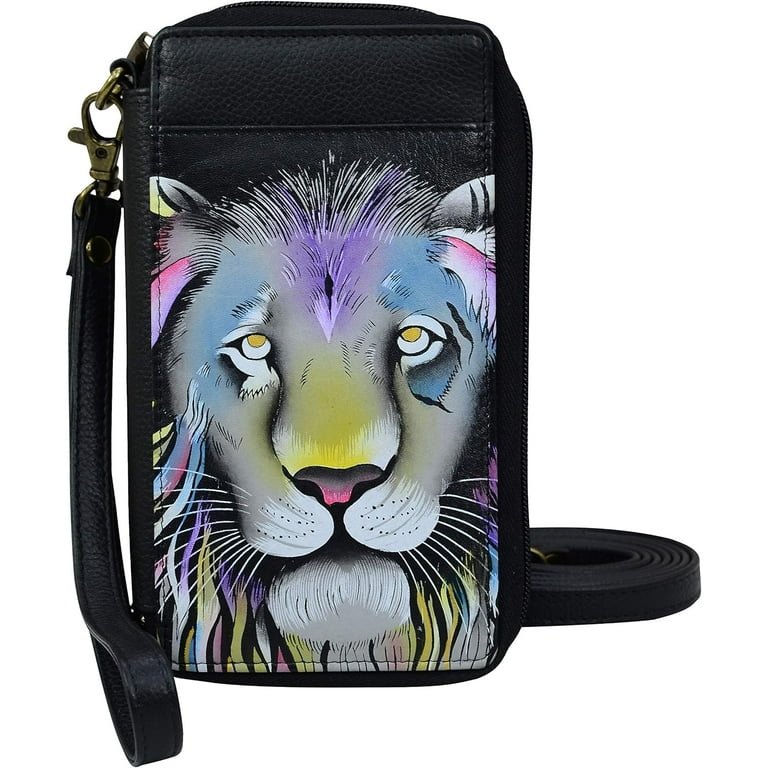This is an image of a small leather wallet set against a blank white background. The wallet, with a faux leather texture, displays an intricate, tie-dyed image of a lion on its front. The lion features a predominantly gray hue with vibrant splotches of blue, purple, pink, and yellow, giving it a decorative and artistic appearance. The wallet is equipped with a golden zipper and includes two straps: a coiled leather strap on the right-hand side and a shorter strap on the left, which has a gold rivet for additional detailing. The right strap is long enough to serve as a crossbody, transforming the wallet into a versatile accessory. The left strap can function as an attachment for a belt or as a wristlet, adding to its practicality.